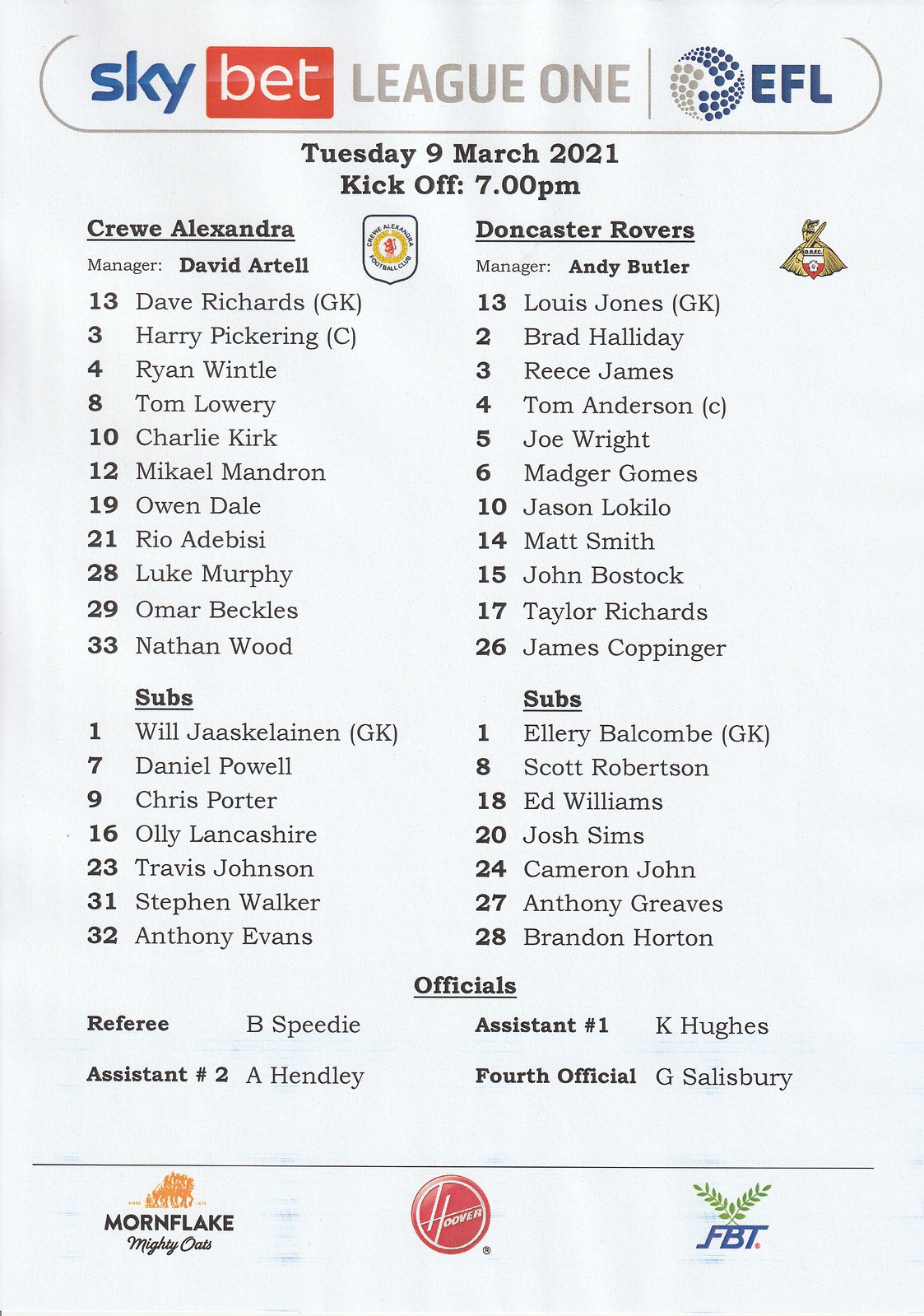This image depicts a detailed flyer for a football match in the Sky Bet League One EFL. At the top of the image, the text reads: "Sky Bet League One EFL, Tuesday, 9th March 2021, kickoff 7 p.m." Below this, there are two columns listing the team members, managers, and logos for Crew Alexandra and Doncaster Rovers. Crew Alexandra is managed by David Artel, and their logo is situated beside their team list on the left side. Doncaster Rovers, managed by Andy Butler, have their team list and logo on the right side. Each column includes player names, numbers, and a section for substitutes. Beneath these player lists, there are the names of the officials for the match, including referees and assistants. At the very bottom of the flyer, sponsors such as Mournflake, Mighty Oats, Hoover, and FBT are listed. The image features a range of colors including white, black, gray, yellow, red, blue, tan, green, and orange, with the layout predominantly centered around black and white text. The overall style suggests a pre-game lineup announcement for the anticipated soccer match.